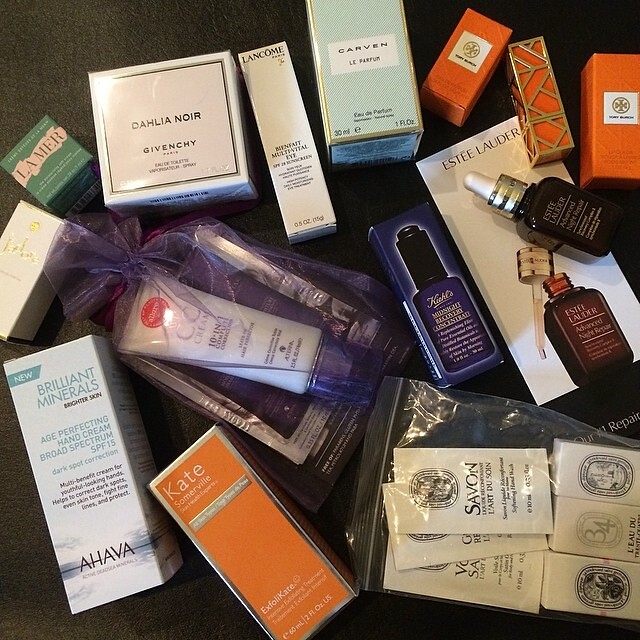This top-down photograph showcases an array of beauty products meticulously laid out on a black fabric backdrop, creating a visually appealing and organized presentation. The arrangement forms a perfect square, with equal dimensions on all sides. Starting from the bottom left corner, a white rectangular box prominently displays blue text that reads "NEW BRILLIANT MINERALS Age-Perfecting Hand Cream, Broad Spectrum SPF 15, Dark Spot Correction, Multi-Benefit Cream for Youthful Looking Hands, Helps Correct Dark Spots, Even Skin Tone, Fight Lines, and Protect." The product's logo, "AHAVA," is clearly printed at the bottom in bold letters. Adjacent to this box, an orange package with elegant silver text and borders features the brand name "KATE SOMERVILLE." Further to the right, a clear plastic bag contains multiple white pouches branded with "SAVANT" in striking black text. Each product remains in its original packaging, except for one, emphasizing the pristine and untouched condition of the items.